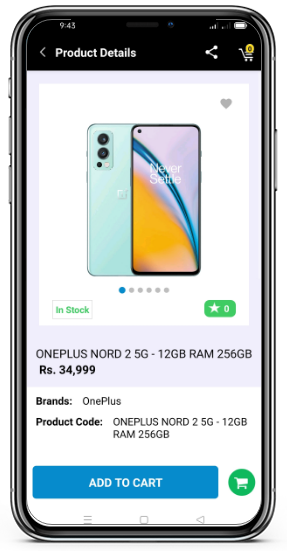The image features a detailed screenshot of an online product page displayed on a black cell phone, showcasing the OnePlus Nord 2 5G smartphone. At the very top of the screen, the title "Product Details" is prominently displayed beside an icon of a triangle with rounded white circles at each corner. Adjacent to it is a shopping cart emblem. Below this header section, the product image is centered within a white square, displaying both the front and back views of the OnePlus Nord 2 5G. The back of the phone is light aqua, highlighting the camera module, while the front screen shows a vibrant mix of orange, dark blue, purple, and creamy white colors, featuring the slogan "Never Settle."

The product description indicates the item is in stock and provides the model details: OnePlus Nord 2 5G with 12GB of RAM and 256GB of internal storage, priced at ₹34,999. The brand name "OnePlus" and the product code "OnePlus Nord 2 5G, 12GB RAM, 256GB" are listed below the price. At the bottom of the screen, there is a prominent green "Add to Cart" button accompanied by a small cart emblem in a green circle.